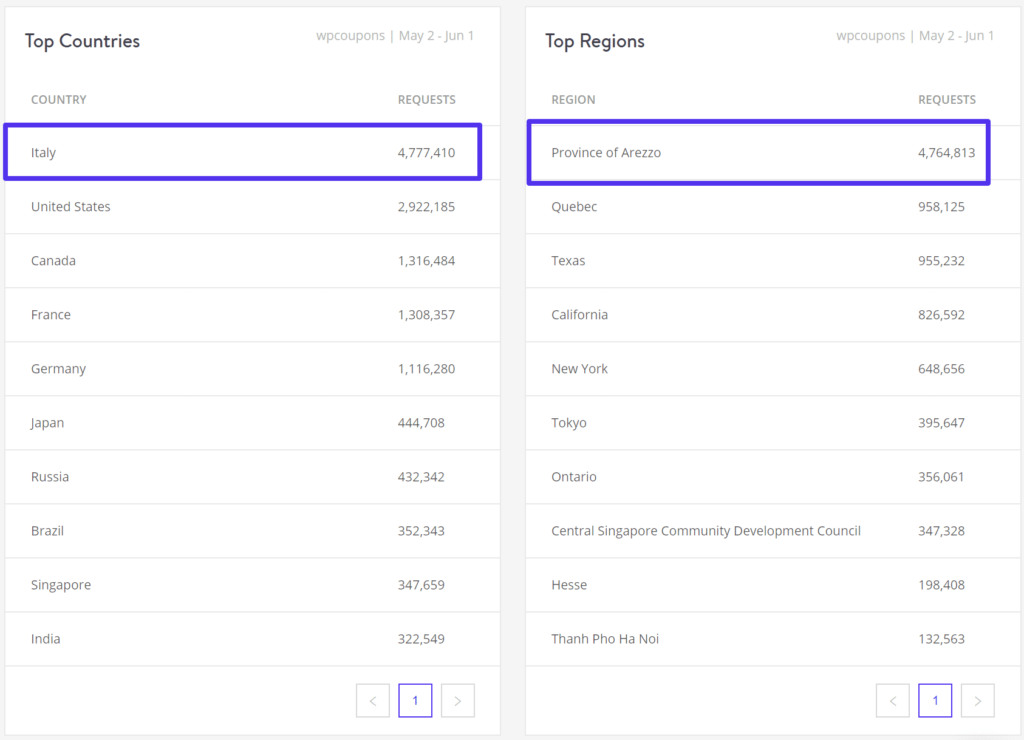In this image, there are two adjacent screenshots displayed against white backgrounds, each featuring black titles with subsequent dark gray text. The left screenshot is titled "Top Countries," while the right one is titled "Top Regions." Both screenshots are from a web page labeled "WP Coupons," covering the date range from May 2nd to June 1st. 

On each screenshot, there are two main columns: "Country" or "Region" on the left and "Requests" on the right. The top item in each list is highlighted with a blue box. For the "Top Countries" list on the left, the highlighted country is Italy, with a request count of 4,777,410. For the "Top Regions" list on the right, the highlighted region is the Province of Rezo, with a request count of 4,764,813.

Following the highlighted entries, the "Top Countries" list includes additional countries such as the United States, Canada, France, Germany, Japan, Russia, Brazil, Singapore, and India. Similarly, the "Top Regions" list includes Quebec, Texas, California, New York, Tokyo, Ontario, Central Singapore Community Development Council, Hesse, and Tan Pho, Hanoi.